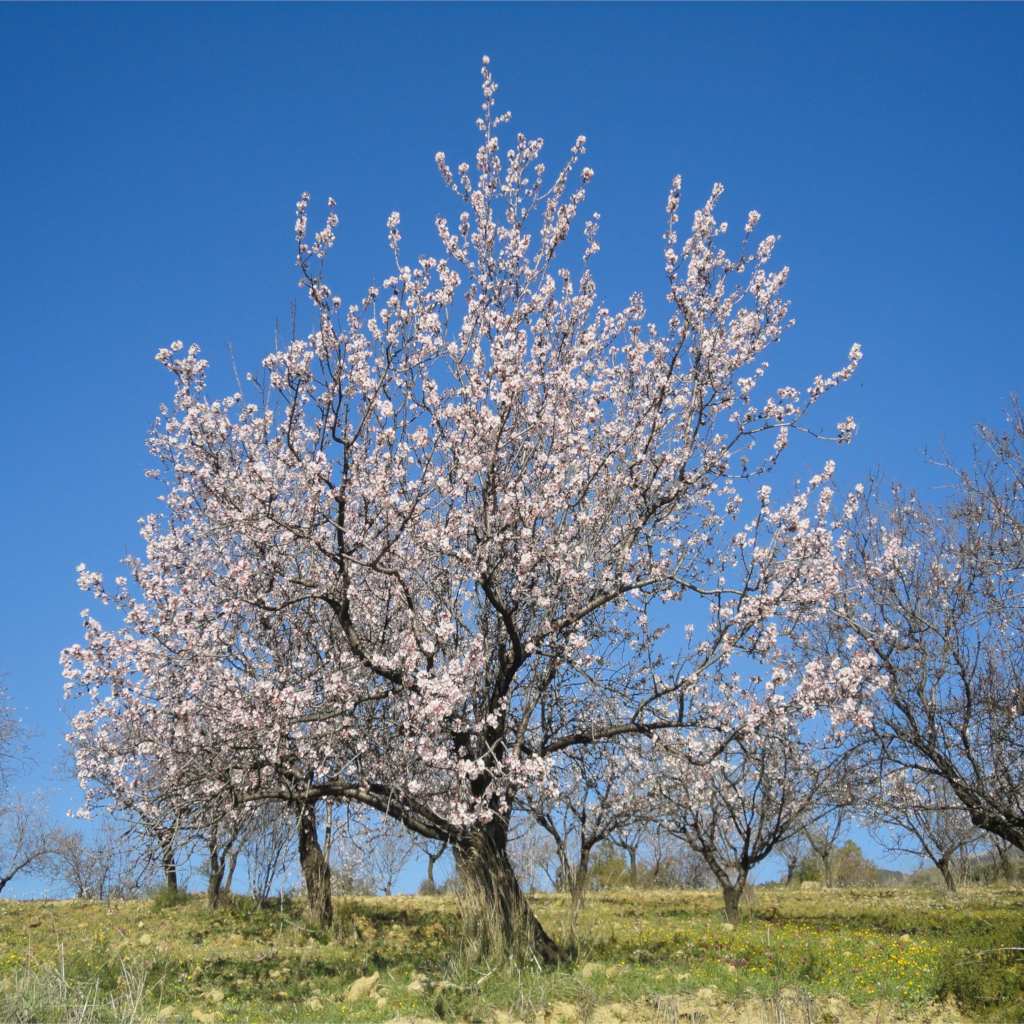This photograph, measuring about six inches square, captures a vibrant outdoor scene during the daytime. The bottom portion of the image is dominated by a sprawling, grassy field punctuated by small yellow flowers and clumps of brown dirt. The grassy terrain stretches upwards from the lower left and right corners, covering approximately three-quarters of an inch before transitioning into the sky. The sky itself is a gradient of blue, darker at the top and lightening towards the horizon.

Central to this image is a lush, prominent tree adorned with an abundance of small white flowers, resembling those of a dogwood or possibly a crape myrtle. This tree, which stands out due to its full and attractive blooming, occupies the majority of the central area. Surrounding it are other smaller trees with thick, dark brown trunks and horizontal branches, also sprouting these delicate white blossoms. 

Overall, the scene presents a serene natural setting with a clear emphasis on the flourishing trees, suggesting an early summer or late spring ambiance under clear blue skies.